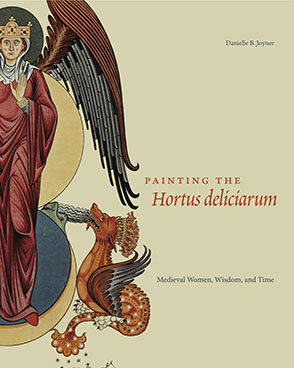The image is the cover of a book, depicted as a vertical gray rectangle. In the upper right-hand corner, in black type, is the author's name, Danielle B. Joiner. Dominating the center, in large red capital letters, the title reads "PAINTING THE" horizontally, with "HORTUS DELICIARUM" displayed beneath it in similarly red but slightly more ornate letters. Towards the bottom, in smaller dark print, the subtitle "Medieval Women, Wisdom, and Time" is inscribed. 

The left side of the cover features a regal figure adorned in a flowing maroon robe, which cascades down to their feet. The figure has a white textile draped around the head and neck, topped with a golden crown encrusted with blue and red gemstones and adorned with gold crosses. Emanating from their left shoulder is a maroonish wing with a gray interior. Their left hand is shown with the palm facing forward, while a substantial part of the right side of their body is cut off by the image's edge. Behind the figure, three concentric circles in gray, tan, and blue hues create a striking backdrop.

At the feet of the figure, an orange dragon with wings is seen, seemingly breathing black smoke towards the robed individual. The dragon faces left, its mouth agape with something gray and white extending out. Notably, the dragon also sports a crown, and its long tail snakes to the left and downward.

Together, these elements form a rich, detailed, and visually compelling book cover that emphasizes its historical and fantastical themes.